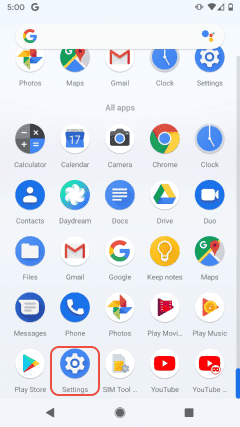This image appears to be a detailed screenshot of a smartphone's home screen or app drawer. At the top, there is a prominent "5G" indicator, alongside icons representing Wi-Fi signals and a half-filled battery. Below this, the Google search bar features a big "G" icon, accompanied by the Google Assistant button.

The main screen is populated with various app icons, including Maps, Gmail, Clock, Settings, and Calculator, featuring symbols for subtraction (minus), multiplication (x), addition (plus), and equals. There’s a Calendar app identified by a blue square, alongside the Camera, Chrome, and Contacts apps. Additional icons include Daydream, Docs, Drive, Duplo, Files, Google Keep Notes, and Google Maps.

Messaging apps are represented, with messages and potentially iPhone messaging icons. Media apps visible include Photos, Play Movies, Play Music, and the Play Store. There are standard utility apps like Settings and a SIM Tool, as well as entertainment and social apps such as YouTube. At the bottom of the screen, there are navigation icons including a left arrow for back, a center button, a square for app switching, and a scroll function, indicating various interactive elements and diverse app functionalities available on the device.